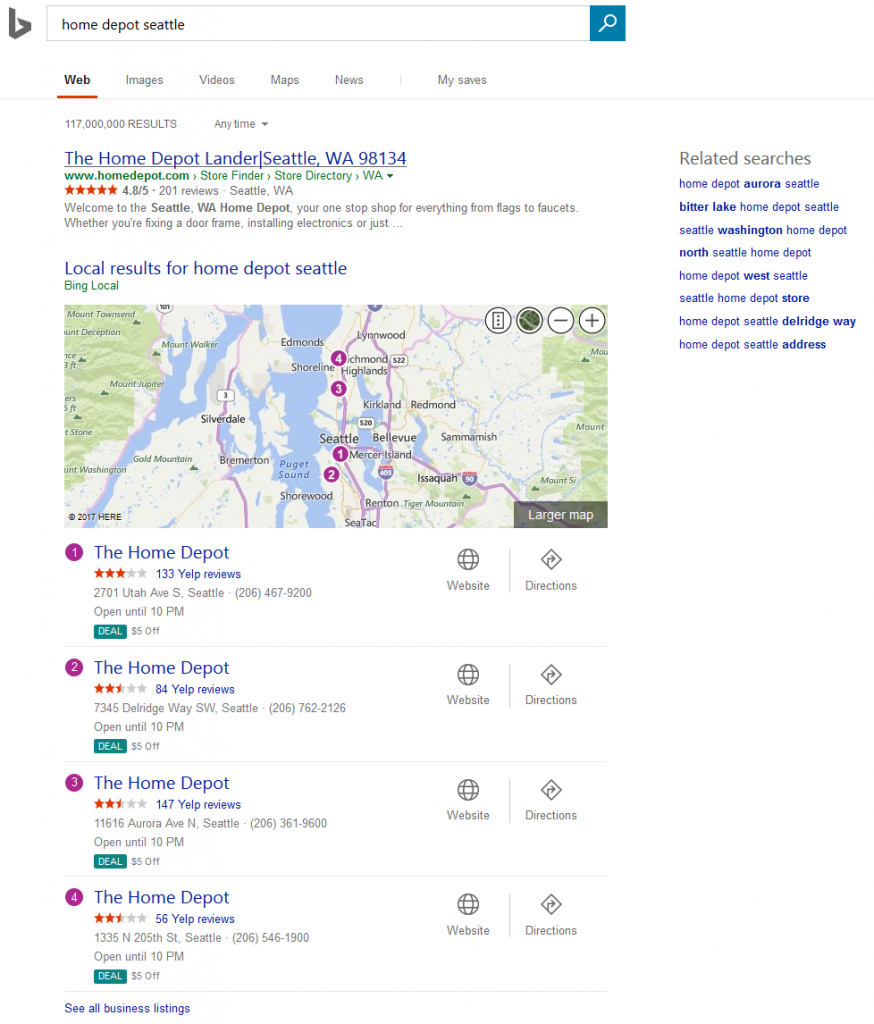The image shows a Bing search results page for the query "Home Depot, Seattle." The search bar at the top displays the repeated search terms "Home Depot, Seattle." Below the search bar, it indicates there are approximately 117 million results. The first search result highlights the Home Depot location in Seattle, Washington, with the address 98134 and a link to www.homedepot.com. This result includes a brief description welcoming users to the Seattle Home Depot, which offers a wide range of products and services, from flags to faucets, and mentions activities like fixing a door frame and installing electronics.

Additionally, the page presents local results pinpointing various Home Depot locations near Seattle on a map. The map features several geographical markers, including Gold Mountain, Mount Jupiter, Mount Walker, Edmonds, Lynnwood, Shoreline, Issaquah Highlands, Kirkland, Redmond, and Sammamish.